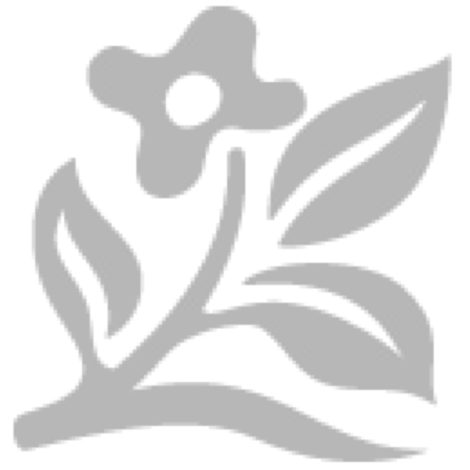This detailed photograph portrays a diverse array of plants, seemingly taken during the daytime in an outdoor setting that resembles either a garden or a forest, perhaps indicating the onset of fall. Dominating the foreground is a variety of bush with leaves transitioning to reddish-brown hues while others remain bright green and tightly clustered. Intermixed are ferns showing signs of browning, suggestive of seasonal change. Nestled behind the ferns is a notable hosta plant, identified by its dark green leaves with striking white edges.

In the background, larger green leaves with light green peripheries mark different plant species. The overall scene is a rich tapestry of leaf shapes and colors, framed by a moss-covered boulder. The ground appears relatively undisturbed, though in need of some care, with visible soil and scattered sticks. This image, devoid of any textual elements, captures a picturesque moment of natural abundance and subtle transition.